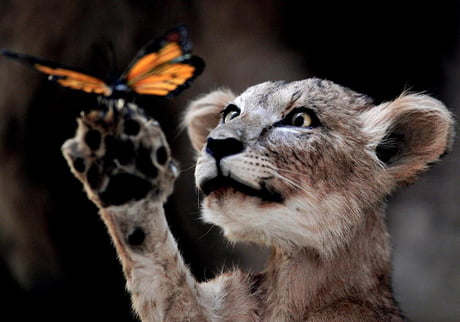This captivating image portrays a young tiger, its wide, alert yellow eyes focused intently on a butterfly perched delicately on its raised right paw. The tiger, featuring a coat of brownish-gray fur interspersed with white around its mouth and under its chin, stands out against a dark background. It has small ears and white whiskers, with black spots near its nose and black markings under its nose and at the start of the fur around its mouth. The tiger's paw, raised in a playful and whimsical gesture, showcases black pads and white fur. The butterfly resting on its paw is striking, with orange wings outlined by a black rim. The overall scene exudes a sense of curiosity and stillness, capturing a rare, serene interaction between the young tiger and the butterfly.